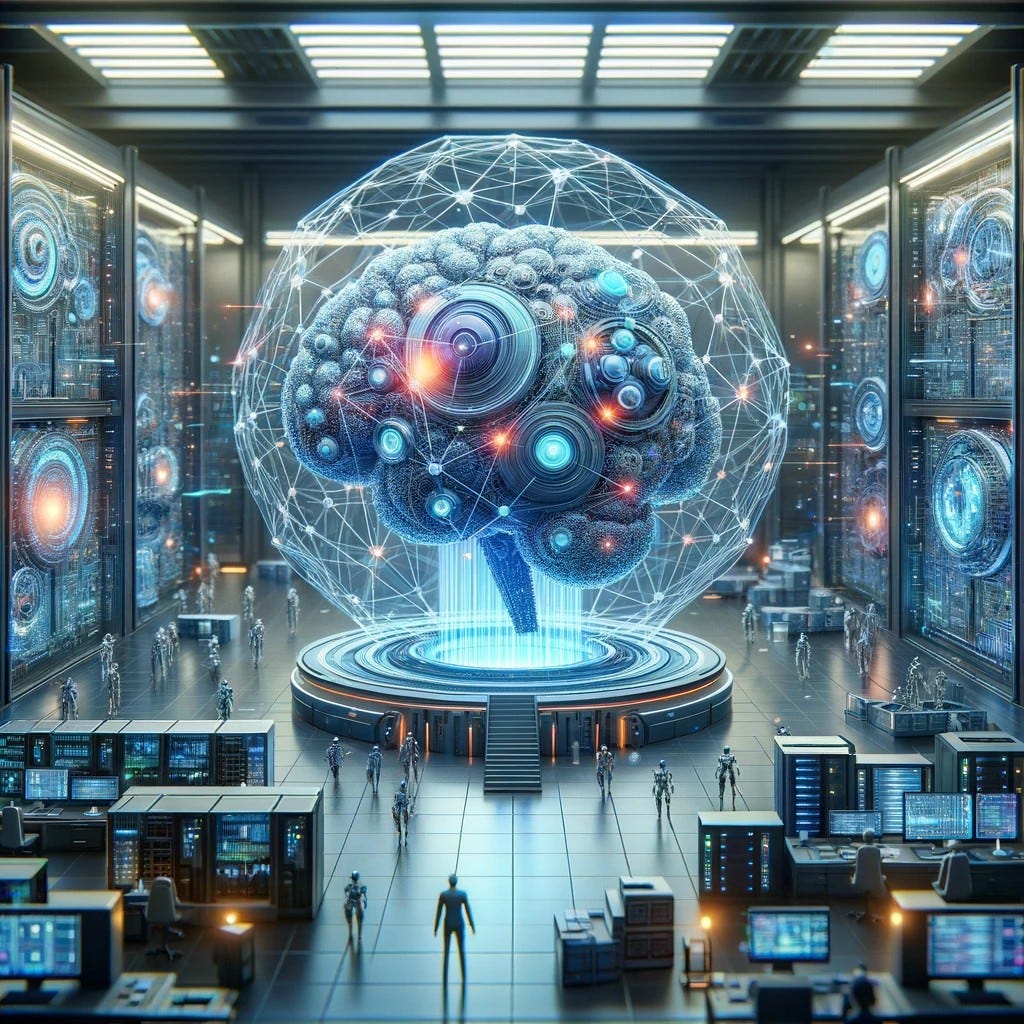In this detailed, computer-generated artwork, we are situated in a vast server room characterized by its digital aesthetics dominated by blues and grays, interspersed with occasional hints of yellows and oranges for illuminated details. The expansive room houses several towering computer servers positioned at the bottom left, bottom right, and along the walls, reinforcing the sense of an advanced computational hub.

At the center of this high-tech environment, a holographic display of a brain augmented with cybernetic enhancements floats majestically. The brain, rendered in shades of blue, features intricate layouts including structures resembling the hypothalamus and is adorned with concentric circles and bright blue lights that illuminate the neural connections. It is encased in a transparent network characterized by dotted, luminescent lines, adding depth to the visual complexity.

Beneath this floating brain, a circular machine projects the hologram upward, and a staircase ascends toward it, providing access to the focal point of the room. Flanking this central machine are robotic figures, systematically organized on both the left and right sides, their attention fixed on the brain hologram. Amidst these robots stands a solitary human figure, positioned at the bottom center of the image, also captivated by the futuristic brain display.

The background is rich with additional technological details; the left and right walls feature displays that seem to showcase galaxies or neural networks, while the back corners house stacks of boxes with circuit-like patterns, particularly abundant on the right and scattered also on the left. This meticulous composition, with its harmonious balance of elements, crafts an immersive vision of a cybernetic nexus centered around the enchanting holographic brain.